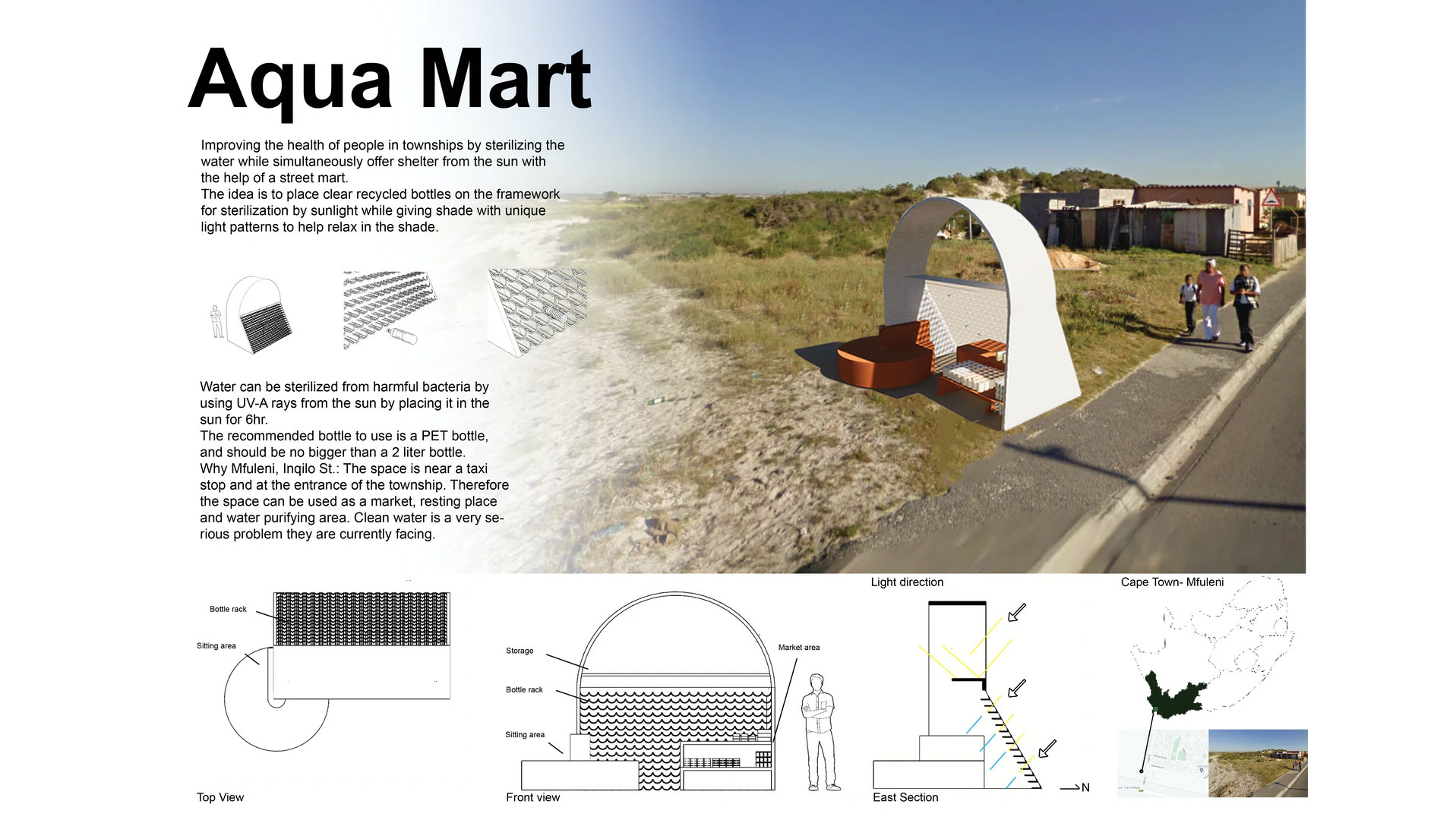The image is a detailed advertisement titled "AQUA MART," with the "A" and "M" capitalized. The central feature is a white and brown circular structure that's open on one side, situated in an outdoor setting with a blue sky and green grass. A sidewalk runs alongside the structure, where three people are visible: a man in a red shirt and white pants, a little boy in dark pants, and a female figure in black pants and a whitish shirt possibly carrying a backpack. Behind the figures, there are several buildings.

On the left side of the image, the text "AQUA MART" is prominently displayed, followed by two substantial paragraphs of black text interspersed with small black-and-white drawings and renderings of the structure. These drawings help illustrate various details and perspectives of the white structure on the right side of the image.

Below these paragraphs, there are three more detailed renderings of the structure, with a highlighted map depicting a country in black next to them. In the lower right-hand corner, a smaller version of the main outdoor scene can be seen. The bottom section of the image wraps up with multiple directional images in various colors, all laid over a landscape that includes red, white, and yellow elements.